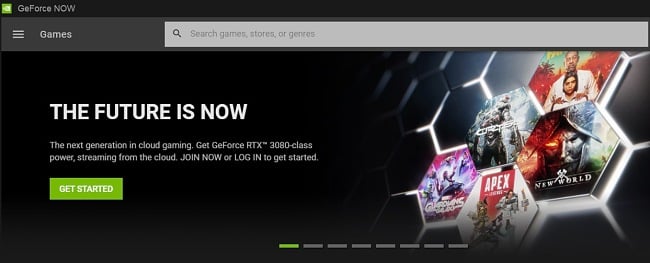The image features a promotional banner for GeForce Now, showcasing advanced cloud gaming technology. The background predominantly features shades of gray and black, with a hamburger menu icon located in the top section. There are various interactive elements, including a search icon designed as a magnifying glass and options to browse games and stories sorted by genre. The tagline "The Future is Now" is prominently displayed, followed by the phrase, "The next generation in cloud gaming," signifying the cutting-edge experience provided by GeForce RTX 3080 class power streaming directly from the cloud.

Below the main text, users are prompted to "Join Now" or "Log In to Get Started." Featured games are highlighted, including "Guardians of the Galaxy," "Crysis," "Far Cry 6," "Apex Legends," and "New World," emphasizing the platform's diverse gaming library. Decorative dash marks add a subtle visual element to the banner, and a series of hexagonal shapes with glowy lights serve as a futuristic background motif. One of the hexagonal shapes appears to be elevated, adding a dynamic layer to the overall design. The imagery and text combined create an inviting and technologically advanced atmosphere, appealing to modern gamers.